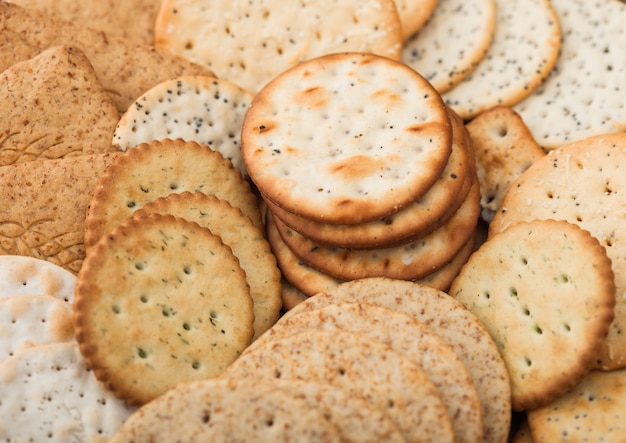This close-up photo showcases a variety of crackers arranged artistically. At the center, there is a straight stack of round crackers, approximately six to eight in number. These central crackers feature a light interior with a golden brown or mildly burnt exterior, suggesting they were carefully baked. Surrounding this central stack, other crackers are laid out in a visually appealing spiral or flower petal pattern. The assortment includes predominantly round crackers, though there are some square ones as well. This mix features crackers with different textures and flavors: some have green herbs scattered throughout, others resemble Ritz crackers with ridged edges, and a few are heavily sprinkled with spices. The crackers vary in color from very white to dark brown edges, depending on their type and baking process. In total, there appear to be around twelve different kinds of crackers, each distinct in shape, size, and flavor, creating a dense and inviting display.